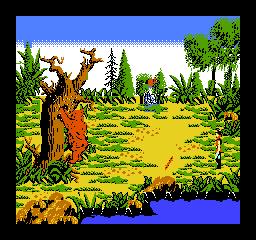In the image, there is a nostalgic representation of an older video game featuring pixelated, cartoon-like graphics. The scene depicts a lush, wooded area predominantly colored in shades of green and yellow, suggestive of a serene forest setting. The bottom includes a patch of blue, likely representing a small pond. On the left side, there is a gnarled brown tree with a bear seemingly digging into a hole at its base, adding a touch of animated wildlife to the environment. Towards the right, a small playable character clad in a brown vest and blue pants stands, poised for adventure. Additionally, another character can be seen in the distance, centrally located within the image. The overall composition exudes an old-school charm, devoid of any text, focusing solely on the vibrant and whimsical forest tableau.